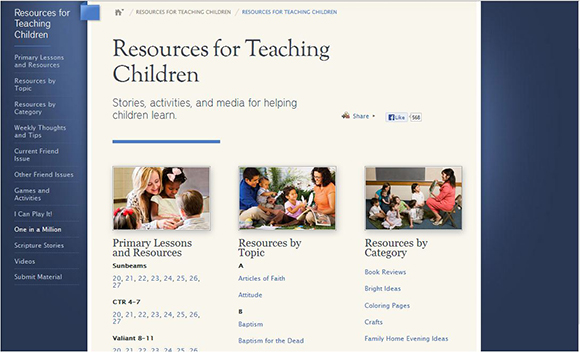The web page serves as a comprehensive resource hub for teaching children. On the left-hand side, a dark blue rectangular sidebar cascades down with multiple sections separated by thin white lines. At the top, bold white text reads "Resources for Teaching Children," adjacent to a slightly lighter blue square.

The following sections in the sidebar are labeled: 
- "Primary Lessons and Resources"
- "Resources by Topic"
- "Resources by Category"
- "Weekly Thoughts and Tips"
- "Current Friend Issue"
- "Other Friend Issues"
- "Games and Activities"
- "IRL"
- "One in a Million" (highlighted in white instead of off-white)
- "Scripture Stories"
- "Videos"
- "Submit Materials"

The main content, set against a tan background, features the title "Resources for Children" in bold black text, followed by a description in regular black text: "Stories, activities, and media for helping children learn." There are Facebook share and like buttons, and beneath are 568 topical entries listed in black text.

A prominent image shows a woman assisting two children with the header "Primary Lessons and Resources." Sections are divided into different age groups: "Sunbeams" in bold black text listing numbers 20-27 in blue, "CTR 4-7" with numbers 20 through 27, and "Valor 8-11" in bold black with numbers 20 through 26.

Another image displays a man in a blue shirt and a woman in an orange shirt next to two children. Below, "Resources by Topic" includes alphabetically-arranged bullet points such as:
- "A: Articles of Faith, Attitude" (both in blue hypertext)
- "B: Baptism, Baptism for the Dead" (both in hypertext blue)

On the right-hand side, another image depicts children in white attire alongside a woman in a red dress and another in a blue dress. The section "Resources by Category" in bold black text lists: 
- "Book Reviews"
- "Bright Ideas"
- "Coloring Pages"
- "Crafts"
- "Family Home and Evening Ideas" (all in blue text).